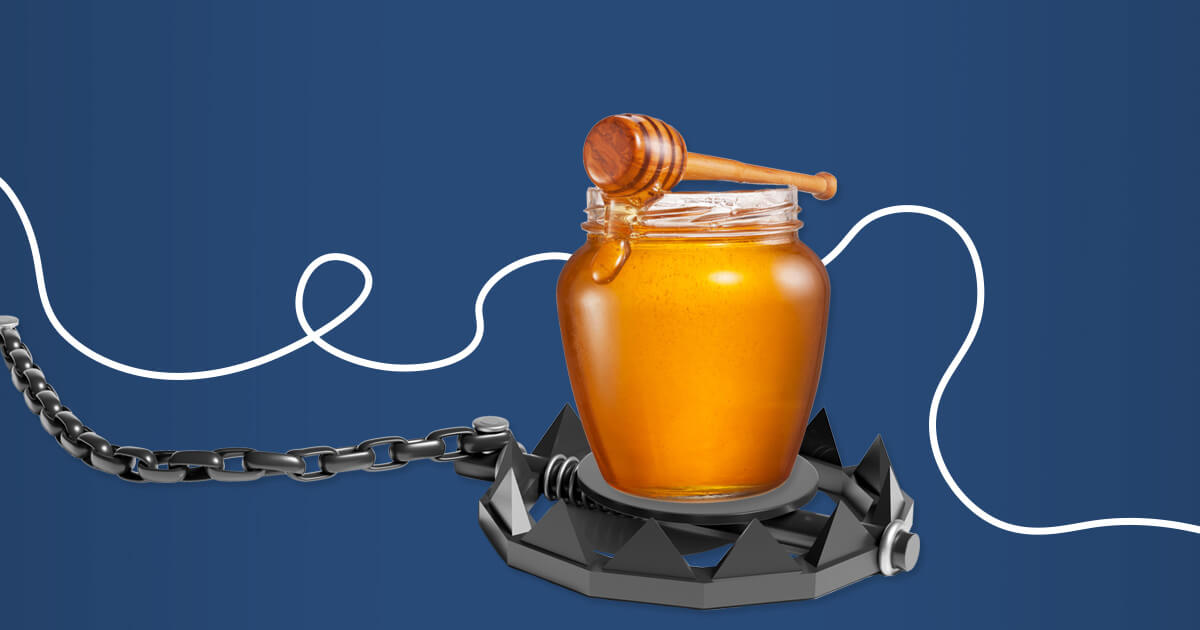The image is a detailed, computer-generated depiction of a large jar of honey prominently displayed against a dark blue background. The honey is contained within a clear glass jar, filled almost to the top with rich, golden-hued honey that is visibly dripping down the side. Perched perpendicularly on the jar is a wooden honey dipper, featuring a beehive design on the broader end, crafted from a mix of brown and darker brown wood.

The jar of honey rests strikingly atop a menacing, dark gray bear trap. This metallic trap is adorned with triangular, razor-sharp points and features a coiled spring mechanism along with silver bolts on its frame. From the trap, a dark gray chain extends towards the left edge of the image, adding to the ominous feel of the setup.

Adding a sense of dynamic motion to the image are swirling white lines that start from the left side and loop elegantly around, eventually disappearing behind the jar of honey and trailing down to the lower right corner. The entire configuration, centered within the frame, creates a striking contrast between the golden honey, the dark, foreboding trap, and the rich blue backdrop.